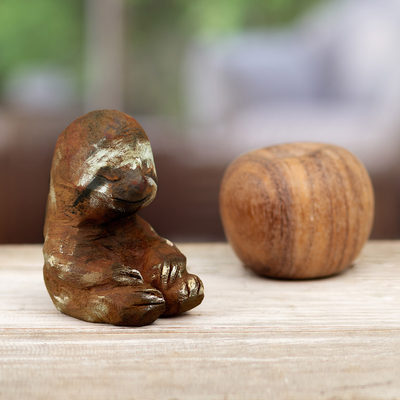A beautifully detailed photograph features a small, wood-carved figurine of a sloth in a sitting pose, with its elongated fingers rested upon its outstretched legs. The sloth's face is painted white with black stripes adorning its cheeks, a brownish face, and a small black mouth. Its eyes exhibit a touch of orange, and the white-painted claws on its hands and feet contrast against the predominantly brownish-orange and subtly white or gray splashes on the body. To the right of the sloth figurine sits a smooth, rounded wooden object resembling an apple with a divot on the top, displaying visible wood grain. Both items rest on a clean, light-colored wooden surface, where the wood grain appears notably large in comparison to the petite sloth and accompanying object. The background features a blurred, white Logan wood parquet area, adding a clean and serene ambiance to the overall composition. The sloth figurine and the apple-like ornament together create a harmonious and aesthetically pleasing visual narrative.